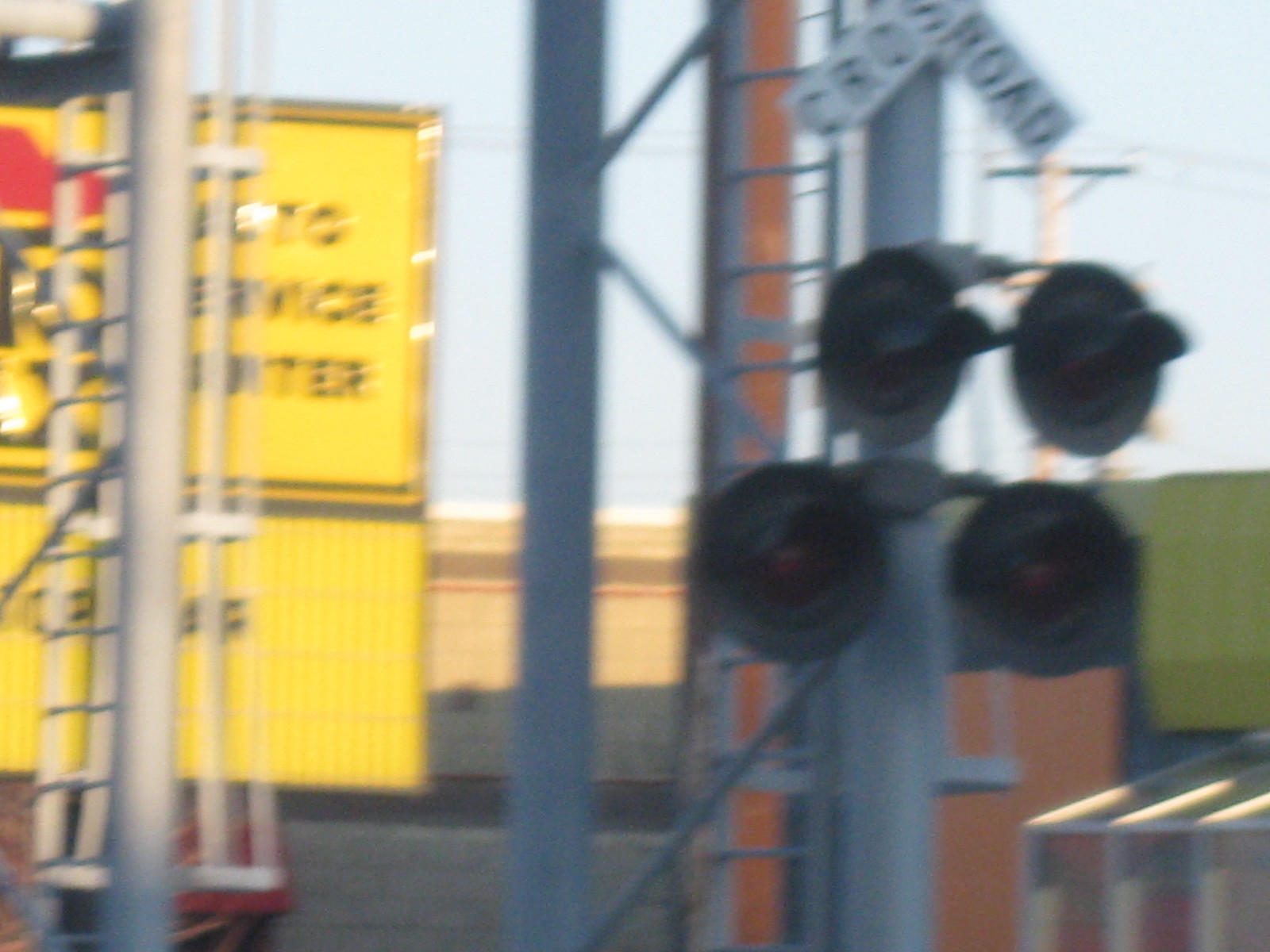This outdoor photograph, though slightly out of focus, captures a multi-layered urban scene centered around a railroad crossing. In the lower right corner, construction studs emerge, seemingly framing a building and anchored to descending posts. Behind this, a vivid green building transitions into an orange structure as the view shifts left. Adjacent to these is a sandstone-colored building adorned with a thick brown stripe near the top and a narrower red stripe beneath it. This building's facade fades into shadow, tinged with gray.

Prominently in the foreground on the right side, stands the railroad crossing, with its distinctive black and white "crossbuck" sign displaying "cross" and "road." The crossing features four signal lights attached to a gray post, which includes a ladder for maintenance access. Additional gray posts support further railroad signals. To the left, another gray post is visible, likely supporting more railroad indicators. A yellow building in the background catches the eye with its bold black lettering spelling out "Service Center." This building also bears red and black signage, partially obscured by the gray post in the foreground.